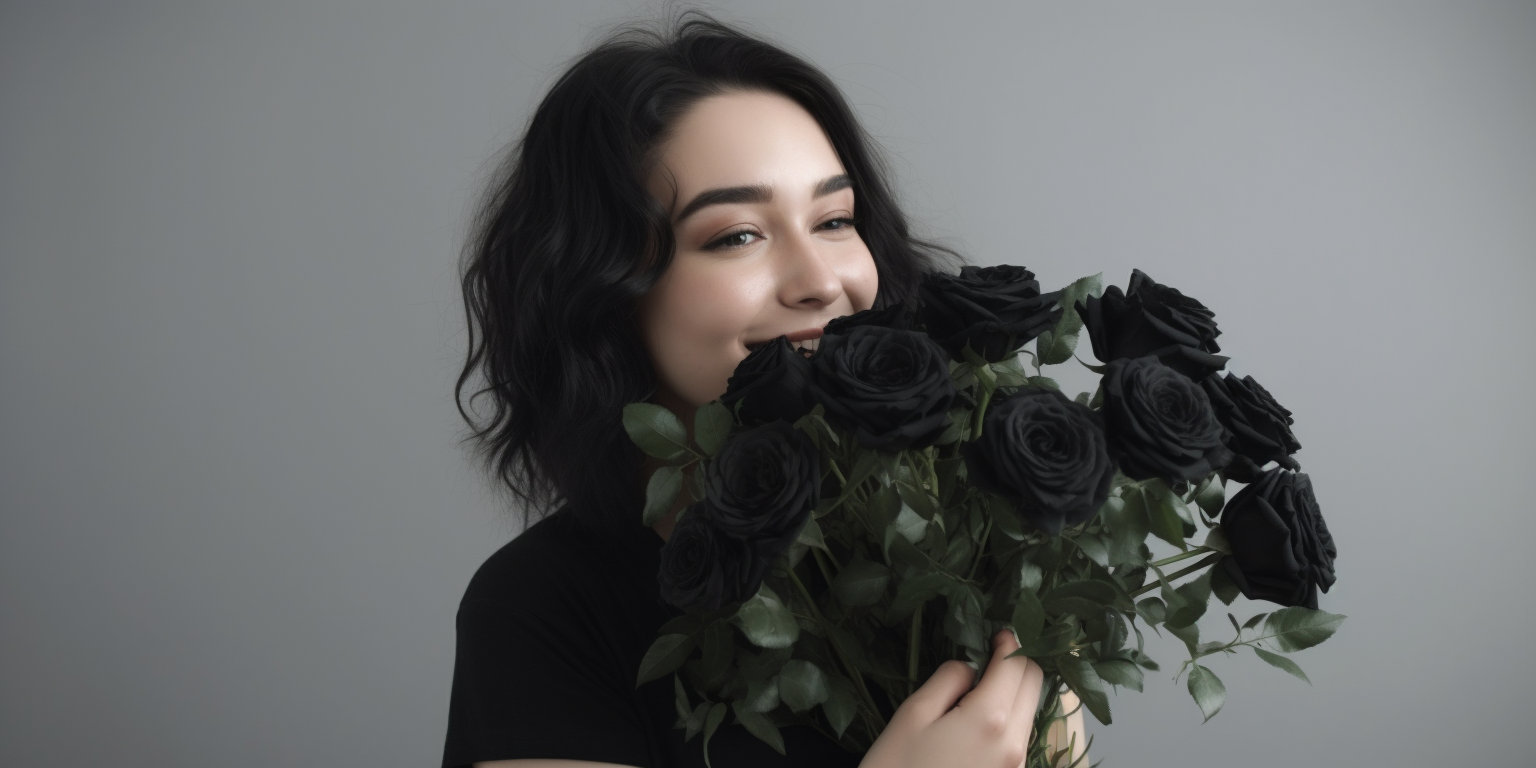The color photograph captures a young, fair-skinned woman with shoulder-length, wavy black hair styled in a bob. She has defined black eyebrows and wears heavy eye shadow. The woman is dressed in a black top, though the sleeve length is not visible as the image only includes her from her shoulders upwards. She is positioned towards the right side of the image and has a large, beaming smile, revealing her upper row of teeth.

Her hands are raised in front of her chest, clutching a bouquet of black-petaled roses. The roses, with their dark green stems and a mix of light and dark green leaves, partially obscure the lower part of her face. The photograph is set against a light gray backdrop that gradually darkens towards the corners, emphasizing her as the central figure. The style of the image is photographic realism, and it is captured in a landscape orientation.